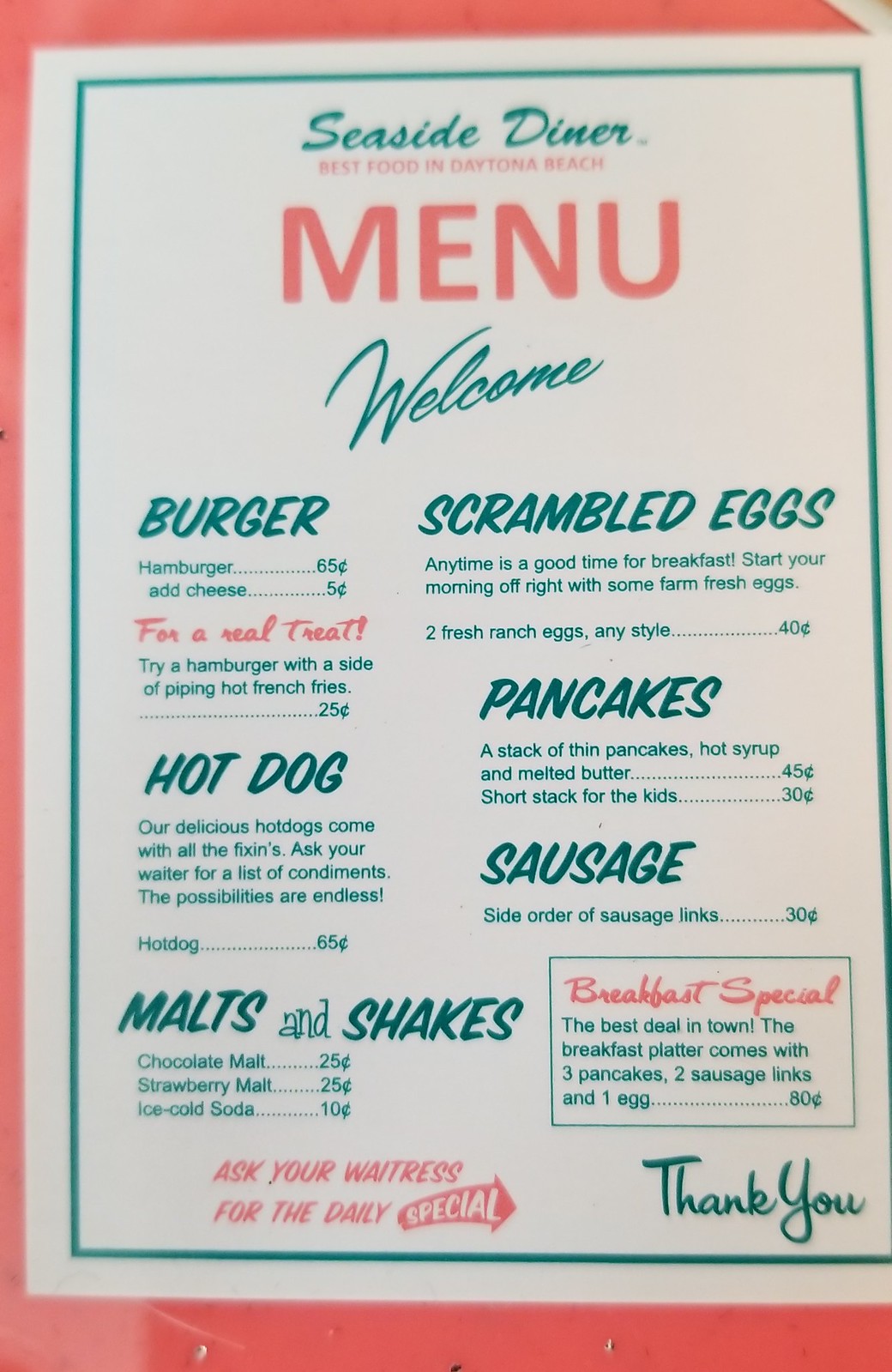**Caption:**

A glimpse into the past at Seaside Diner in Daytona Beach reveals a vintage menu encased with an orange border, hinting at its role more as a nostalgic display than a functional menu. This single page of the historical menu lists classic American diner fare with impressively low prices that suggest it hails from a bygone era. Offerings include a hamburger and hot dog at $0.65 each, two fresh ranch eggs cooked any style for $0.40, and a breakfast platter touted as "the best deal in town," featuring three pancakes, two sausage links, and one egg for just $0.80. Additional delights include a chocolate malt for $0.25 and an ice-cold soda for $0.10. The menu warmly invites patrons to "ask your waitress for the daily special," encapsulating the charm and simple pleasures of traditional diner dining.